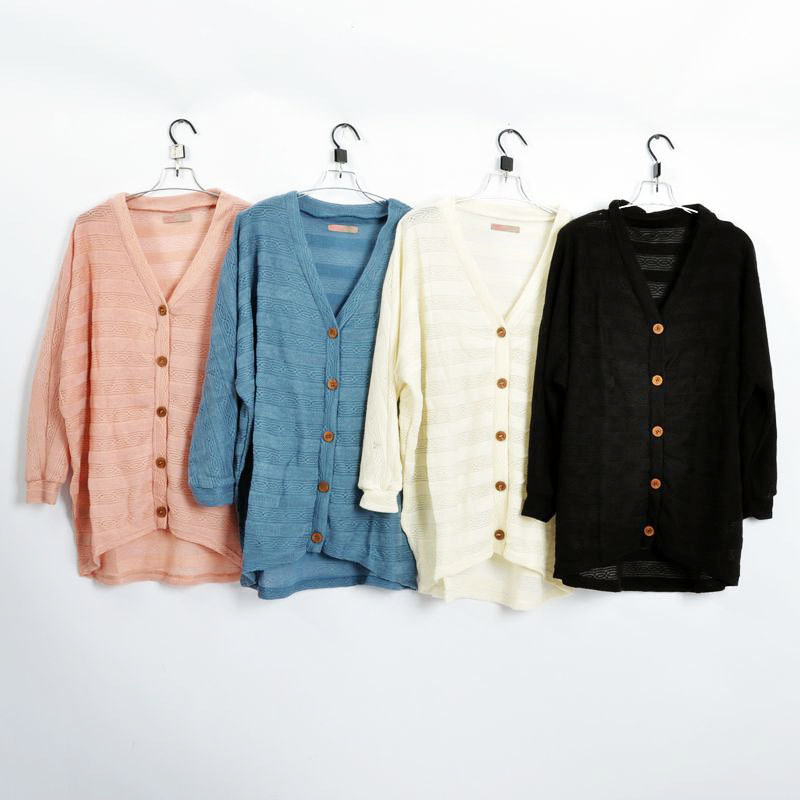The color photograph features four cardigans hung on black hangers, lined up from left to right against a light gray background that appears lighter towards the top. Each cardigan is fastened with five brown buttons down the front, and they overlap slightly. The hangers have darker tops and black hooks pointing to the right and downwards, with the rounded part on the left side.

Starting from the left, the first cardigan is a peach color with an embossed horizontal stripe design and a little blue or white tag at the top. The second cardigan is light blue with lighter blue striping and also features a similar design to the first. The third cardigan is cream-colored, sharing the same design and button pattern. Finally, the cardigan on the far right is black with a black and gray striped interior and a black tag at the top. All cardigans have long sleeves and small, difficult-to-read labels inside the neckline. The background's lighter gradient gives the photograph a soft, cohesive look.